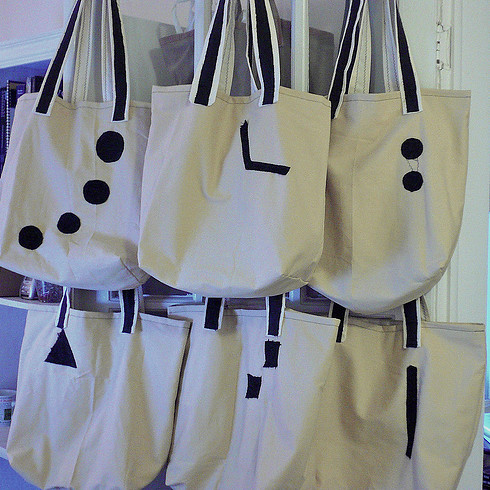This photograph showcases six or seven khaki-colored canvas tote bags arranged along a rack. Each bag features black and white striped handles, with the white stripe on the outside and the black stripe on the inside. Starting from the top row on the left, the first bag exhibits four black dots arranged in a curving line upward. The middle bag presents an L-shaped or 105-degree angle in black on the top right corner. The top right bag features two vertically aligned black dots with a small space between them. On the bottom row, the left bag displays a black triangle at the top left corner. The middle bag has two black squares arranged like descending stairs towards the left. The bottom right bag carries a single vertical black line running from the top towards the bottom. The overall composition focuses on the distinct black patterns printed on each bag against the neutral canvas background.